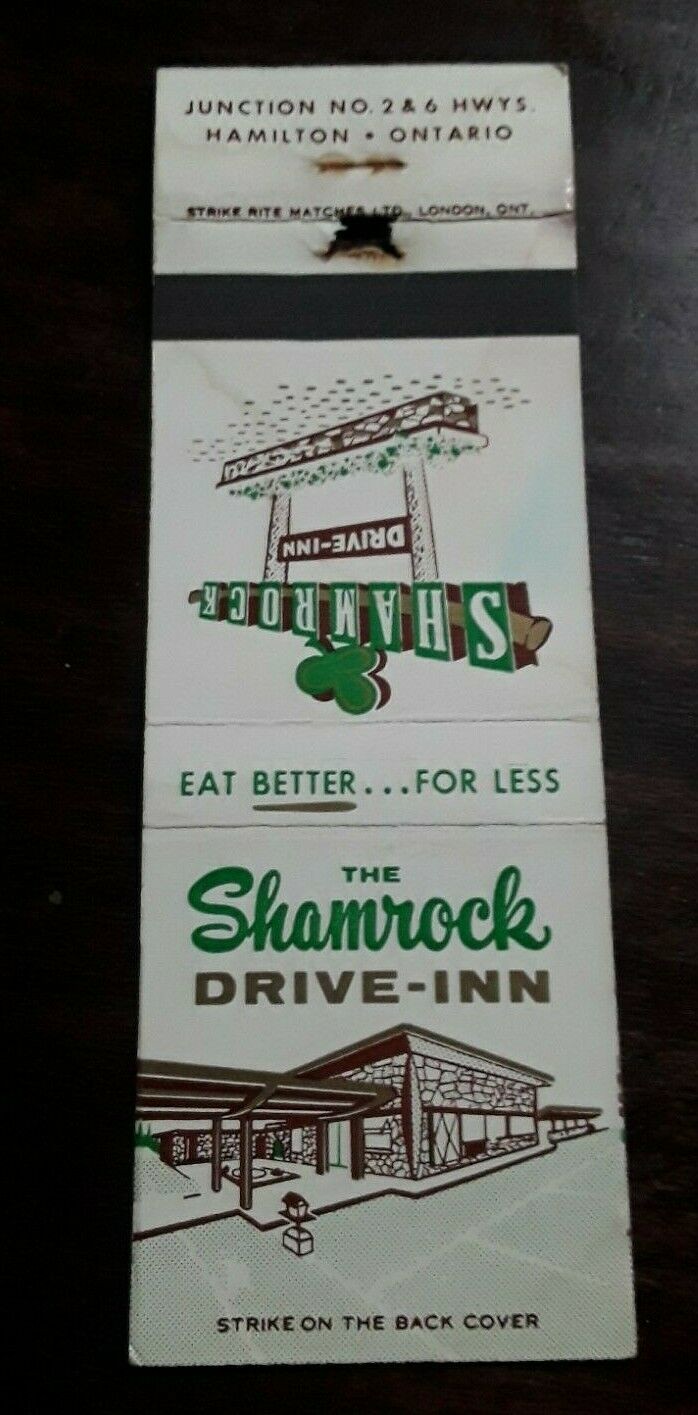This matchbook from the Shamrock Drive-In is fully open, revealing both its front and back covers. The front cover, in a right-side-up orientation, features "The Shamrock" written in a green, brushstroke cursive font. Below, in brown text, it states "Drive-In" followed by an illustration of a one-story building adorned with stonework. The building has an overhead car cover in front of its entrance, surrounded primarily by a parking lot. The tagline "Eat better... for less" is written above in green, with "better" underlined in brown. An instruction reads "Strike on the back cover."

Flipping to the upside-down back cover, each letter in "Shamrock" is encased in its own rectangle, topped by a shamrock illustration. Below the name, "Drive-In" is inscribed in brown between two posts, mounted on a brick planter filled with clover. The upright section details the location: "Junction Number 2 and 6 Highways, Hamilton, Ontario." It also includes the manufacturer details: "Strike-Rite Matches Limited, London, Ontario.” There is a small burnt spot near the "Strike-Rite Matches Limited" text, and the matchbook is set on a black tabletop.